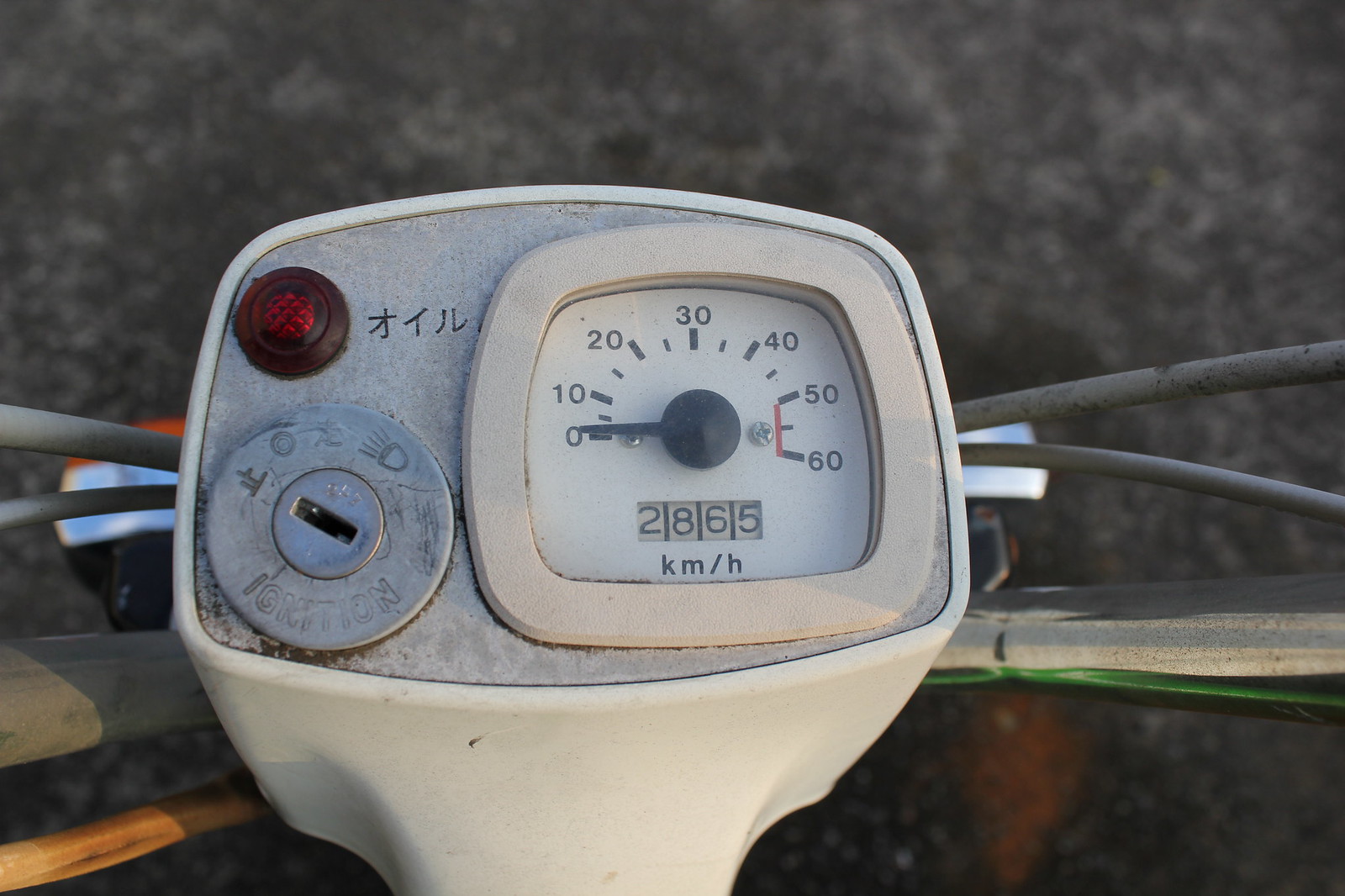This rectangular image, oriented horizontally, features the dashboard and controls of a moped, possibly resembling a Vespa. Central to the picture is the speedometer and odometer, encased in a white frame that also houses the ignition switch and a small red indicator light. The base of this structure is metallic silver, adding a sleek contrast to the white elements. A keyhole is present, suggesting the point of ignition for the moped. Notably, a symbol indicating the headlight switch is visible.

The handlebars extend from the centerpiece, partially visible and leading out of the frame, hinting at the control mechanism for the rider's hands. Various cables, likely related to braking, stem from the base of the speedometer and odometer structure. The background below is a dark gray, resembling concrete, suggesting the moped is stationary and perhaps parked. In the lower-left corner, there is an ambiguous red and metallic object, its purpose unclear from the image. Overall, the photo provides a close-up view of the main controls and structure of a motorized two-wheeled vehicle.